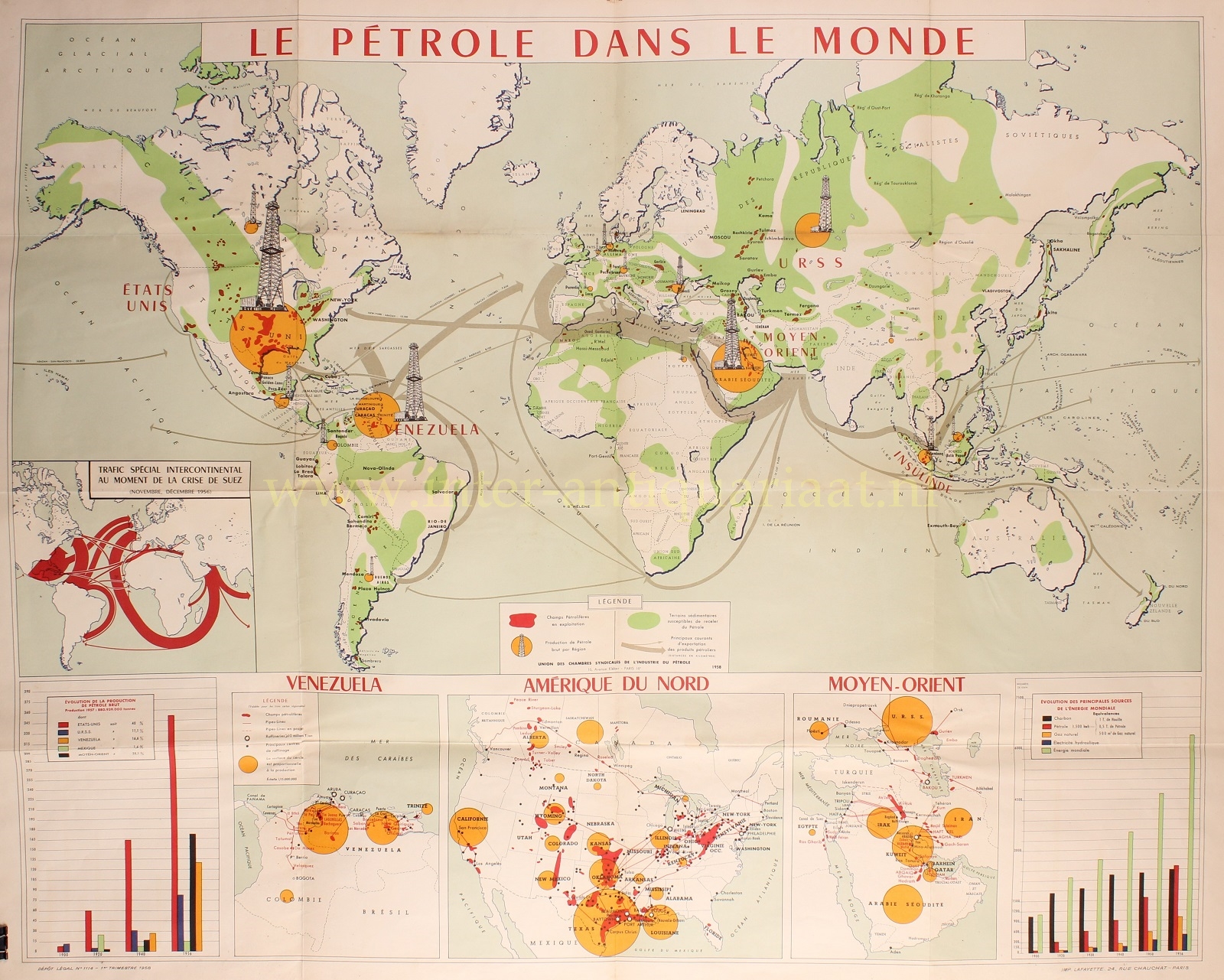The image depicts an older map titled "Le Petrole dans le Monde," showcasing the global distribution of oil. The map covers North and South America, Africa, Europe, Asia, and Australia, rendered in pale hues of white, light gray, light green, and yellow. Prominent yellow circles, each overlaid with images resembling oil rigs, dot various regions, indicating significant oil sites. 

At the bottom of the map, there's an array of informational boxes. The leftmost box features a bar graph, followed by a section labeled "Venezuela" with an inset map highlighting part of the country. Adjacent is another section labeled "Amérique du Nord," though the text is less legible. The next box, titled "Moyen-Orient," is densely populated with yellow circles, reflecting the concentration of oil rigs in the Middle East. The rightmost box contains a different bar graph. The map also includes several legends and charts, presumably providing further insights into global oil distribution and flow, though specifics are hard to determine due to the language barrier. The overall map is punctuated with numerous yellow circles, illustrating the global spread and crucial hubs of oil production.